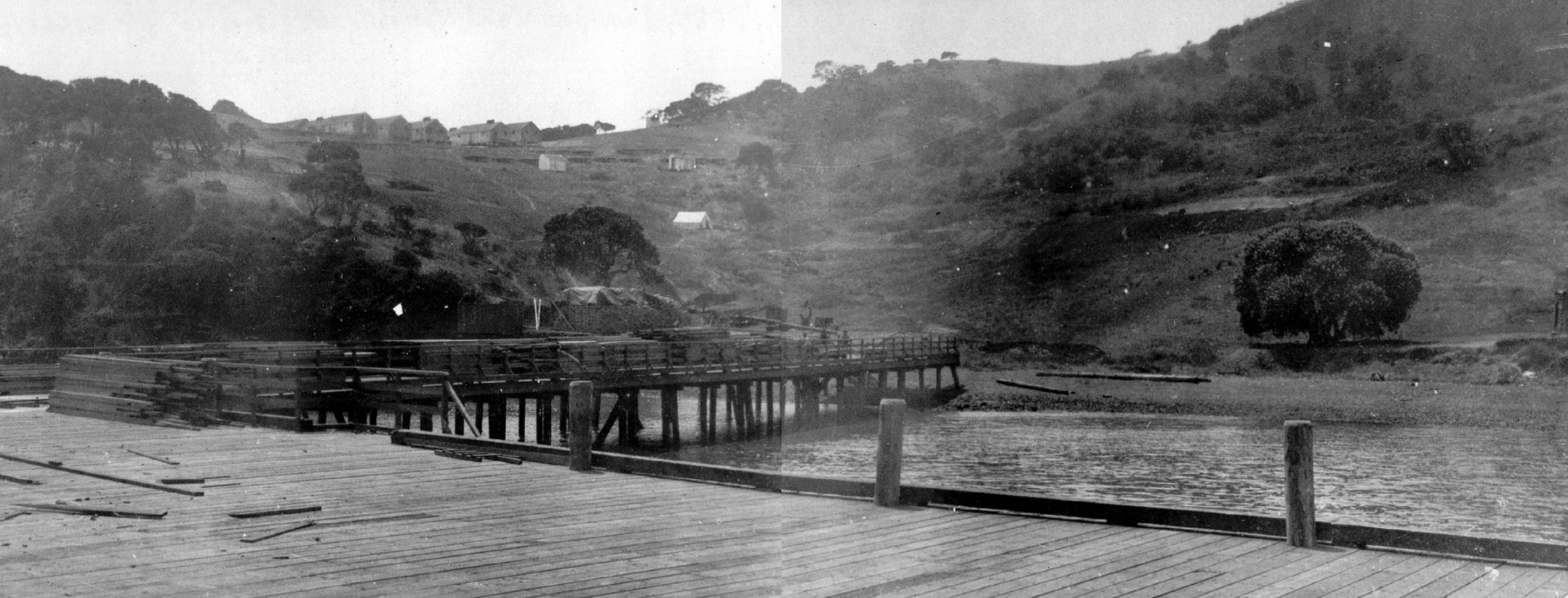This black and white vintage photo, potentially from the 1930s or 1940s, captures a large wooden dock structure extending over a lake. The image, likely composed of two older photos merged together, portrays a spacious dock around 30 feet across, with wooden poles and loose boards indicating possible construction or repair work. In the background, faint outlines of smaller structures—possibly houses—can be seen on steep hills or cliffs. The scene is framed by a tree on the right side and more trees ascending the hillside. The dock appears to be a significant platform, blending into the foreground of the combined images, with a wooden pier extending further into the water. Beyond the dock, the landscape features a body of water, steep hills, and a rugged natural backdrop, highlighting the serene yet aged ambiance of the setting.